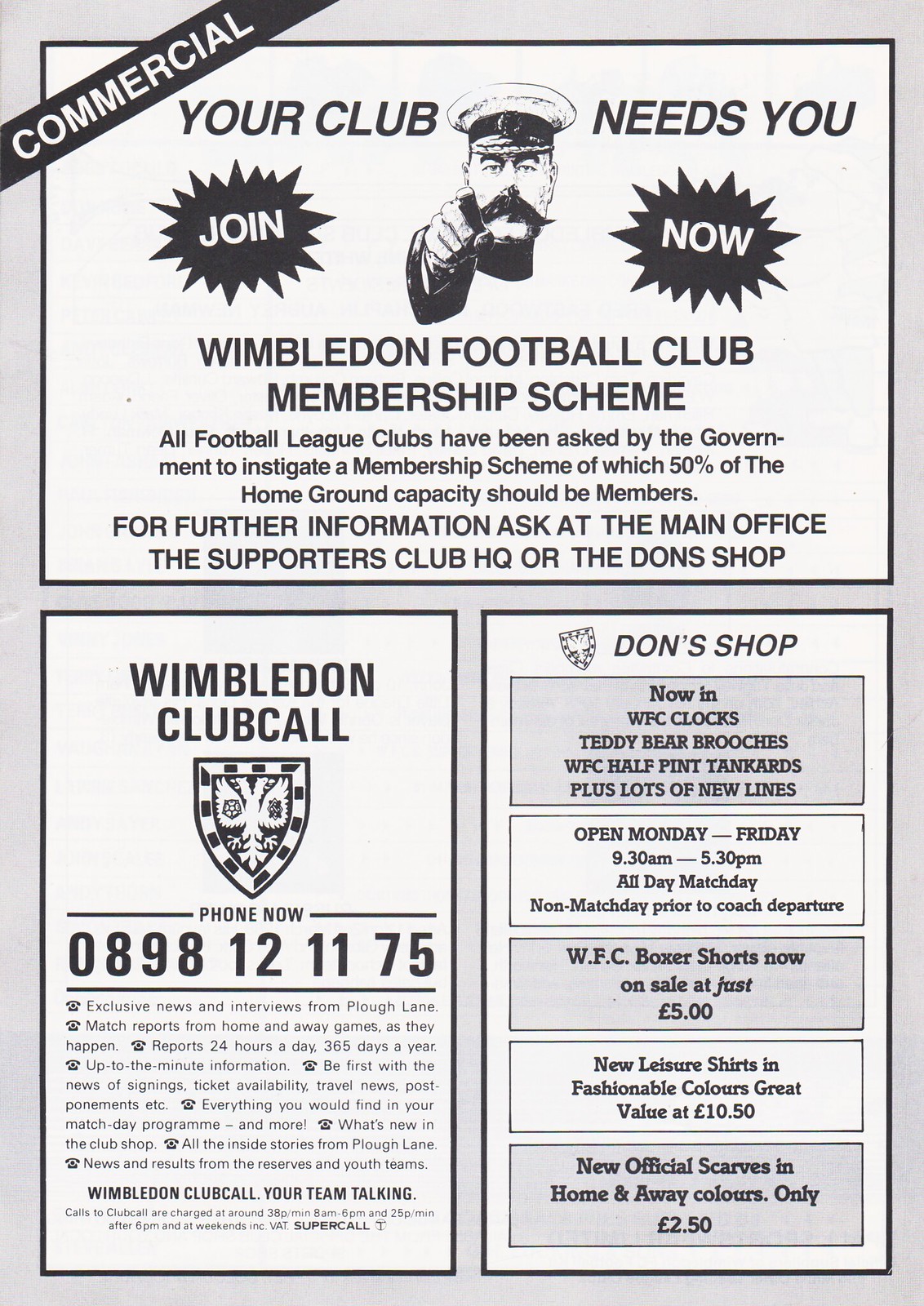This image showcases a vintage black-and-white printed page from a football program, primarily in portrait orientation. The background is light gray, divided into three sections by black borders. The top half prominently features a large white square with a black outline. At the very top left corner, a black diagonal banner reads "Commercial" in large white text. Just below it, the central headline captures the reader's attention with, "Your Club Needs You," displayed above a striking illustration of a man wearing a military cap and sporting a distinctive handlebar mustache, evocative of a historical recruitment poster. This figure is framed by black conversational bubbles with white text; the left bubble reads "Join," and the right one reads "Now."

Beneath the commanding image, the text "Wimbledon Football Club Membership Scheme" appears in bold black print, followed by a smaller paragraph explaining the membership scheme and the directive from the government for football league clubs. For further details, readers are directed to the main office, the Supporters Club HQ, or the Don Shop.

The lower half of the page is split into two vertical advertisements. The left section is titled "Wimbledon Club Call" and includes a SHIELD logo above a contact information paragraph. Meanwhile, the right section is headed "Don Shop," featuring a logo and multiple boxes of information that include phone numbers and operating hours, alternating in gray and white backgrounds.